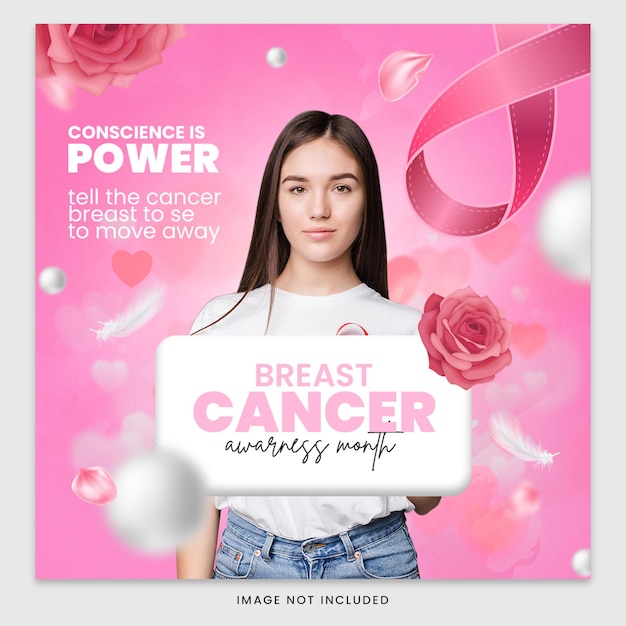The poster for Breast Cancer Awareness Month features a central pink square set against a gray background that forms a large outer border. Within the pink square, the upper left corner showcases a delicate rose, while the upper right corner displays the iconic pink ribbon symbolizing breast cancer awareness. A scattering of petals, white feathers, and small white balls embellishes the background, adding a soft, decorative touch.

At the center of the poster stands a woman with long, dark hair and a pleasant expression. She is seen from the waist up, wearing a white T-shirt and jeans, facing the viewer directly. In her hands, she holds a rectangular sign with curved edges. The sign prominently features the words "breast cancer" in large pink letters, with "Awareness Month" written below it in a smaller black script.

To the left of the woman’s head, bold white letters on the pink background proclaim, "Conscience is Power," with the word "Power" standing out in larger font. Below this, another line in white text reads, somewhat cryptically, "tell the cancer breast to say to move away," with an apparent typo in the word "say," misspelled as "S-E."

At the bottom center of the gray border, in black type, is the disclaimer "image not included."

This visually striking poster combines symbolic imagery and motivational text to emphasize the importance of breast cancer awareness and the empowering message of early detection and action.